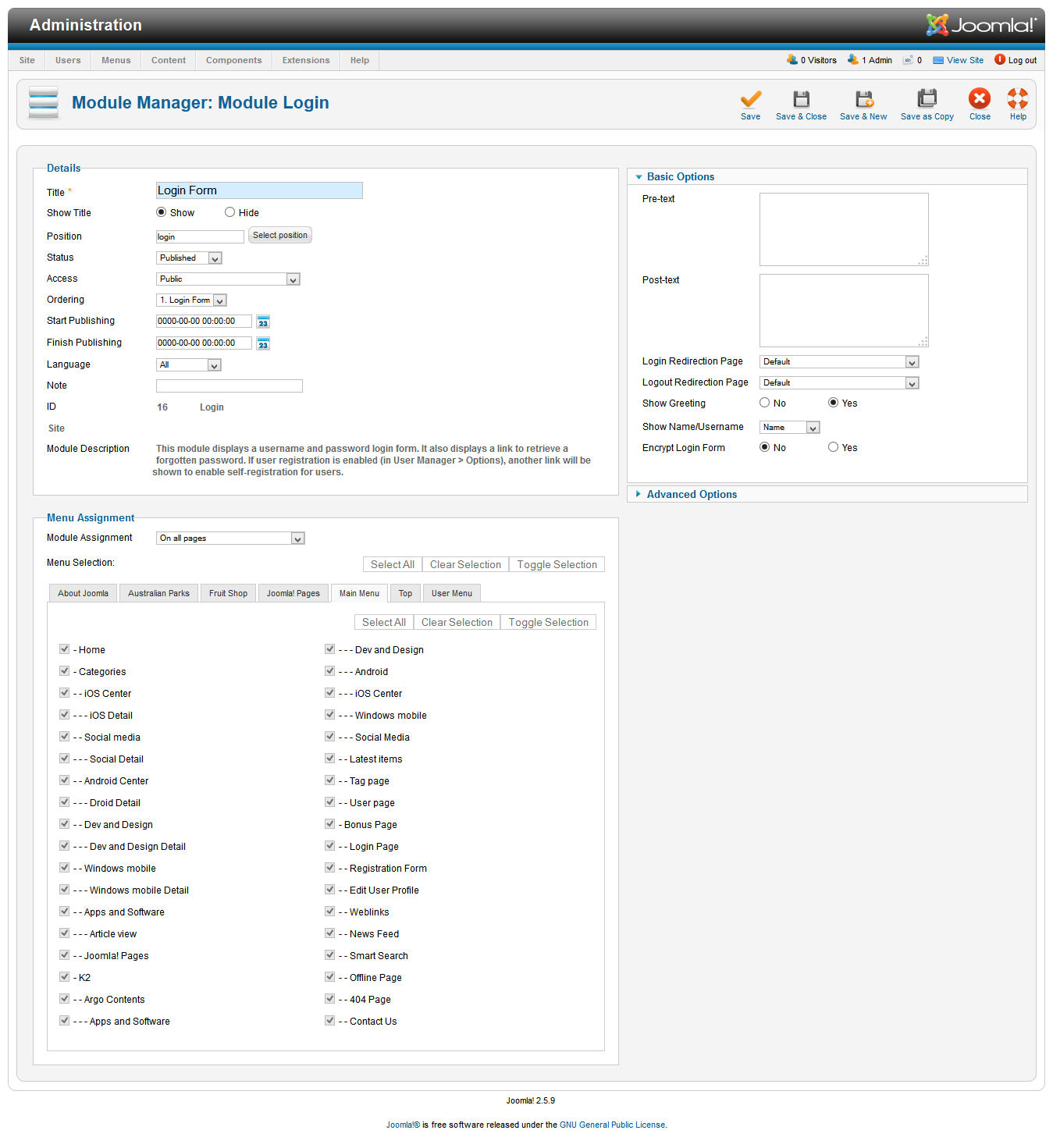### Caption for Joomla Administration Panel Screenshot

This detailed screenshot showcases the Joomla administration panel, highlighting the "Module Manager" section for managing login modules. The page, titled "Joomla", features a black background with white text displayed at the top right. The top left corner identifies the interface as "Administration".

Key tabs across the top include "Sites," "Users," "Menus," "Content," "Component," "Extensions," and "Help." The right side of the panel provides quick stats: "0 Visitors," "1 Admin," and a "Logout" option below that.

On the left, under "Module Manager," the "Module Login" is marked in blue. The right side offers action buttons, including an orange tick for "Save," "Save & Close," "Save as New," "Save as Copy," and a red "X" for "Close."

Within the "Module Manager" section, detailed options are visible:
- **Detail Options:** Title "Login Form," "Show Title," with "Show" selected, and other attributes such as Position, Status ("Published"), Access ("Public"), Ordering ("Login Form"), Start/Finish Publishing, Language ("All"), Note, ID ("16"), and Module Description. The description clarifies that this module displays a login form for a username and password and includes links for forgotten passwords and user self-registration if enabled in the User Manager options.
- **Menu Assignment:** The module is set to display on all pages, with selections including "About Joomla," "Westerland Parks," "Fruit Shop," "Joomla Page," "Main Menu," and "Top User Menu." It covers various menu items and categories like "Home Categories," "iOS Sense," "Social Media," "Android Sensor," "Dev and Design," "Windows Mobile," "App and Software," "Article View," "Joomla Page," "K2," "ARCO Content," among others, all of which are checked.
- **Basic Options:** Fields for "Pretext," "Post Text," redirection options for login, and visibility settings for greetings and usernames, names, and login clicks.
- **Advanced Options**: Listings for further customization.

The panel serves as a comprehensive interface for website administrators to manage user login modules and assignments efficiently within the Joomla platform.